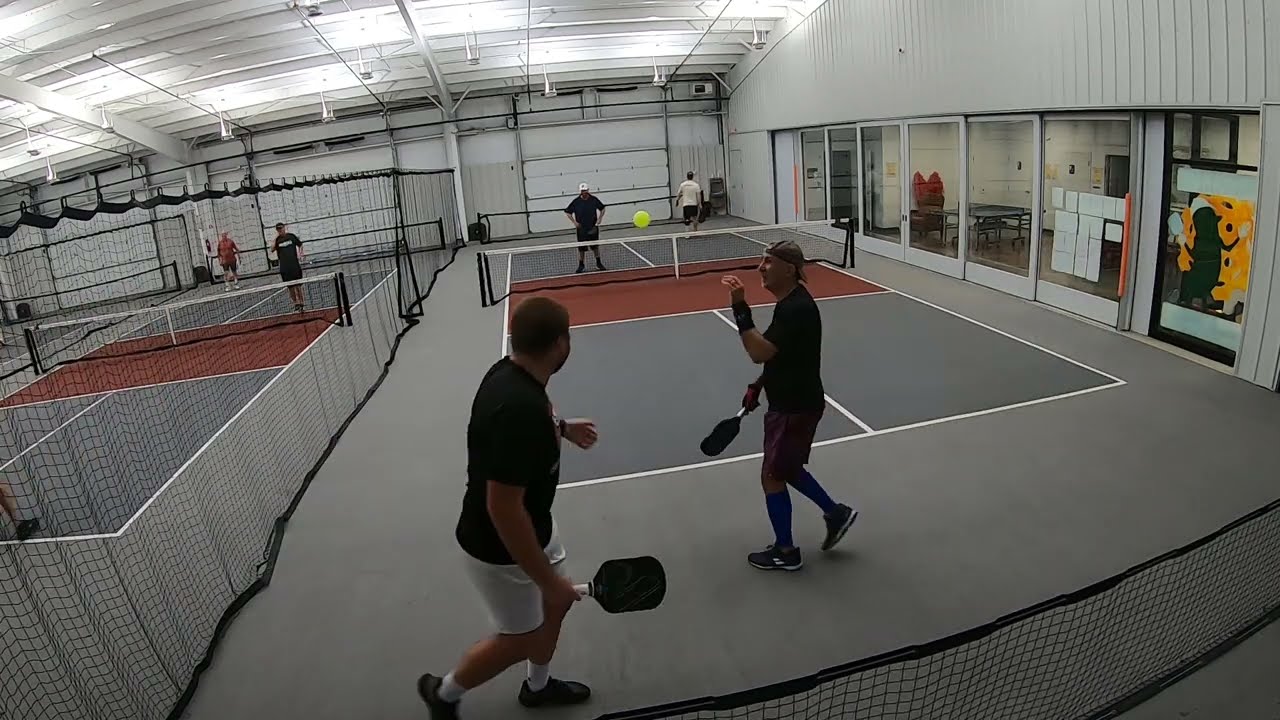The image depicts an indoor sports center housed within a metal Quonset hut-style building, marked by exposed beams and fluorescent lighting. The main focus is a dark gray court outlined with white paint lines, featuring a low net, about waist-high, suggesting the sport of pickleball. Two men are actively engaged in a doubles game, wielding rectangular, solid black paddles and playing with a white ball. Both players are dressed in athletic gear, with short-sleeved shirts, shorts, and sports shoes, one notably wearing a backwards hat. Adjacent to them, there's a glass-paneled spectator area, and another identical pickleball court is visible to the left, separated by a mesh curtain. This second court also features players practicing. The gym floor overall is a lighter shade of gray compared to the courts, and the space is dominated by white walls and ceiling. A ball is suspended mid-air in the center of the image, possibly at the moment of serve.